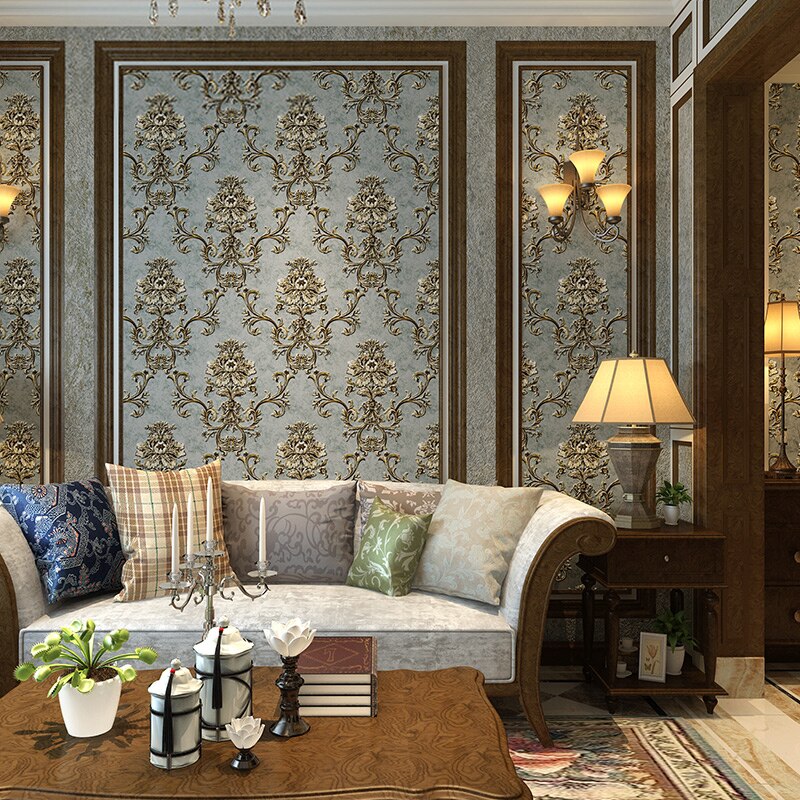This detailed photograph captures a richly decorated, square-shaped living room with a dramatic blue and gray floral wallpaper adorning the back wall. The wallpaper features an intricate, busy design with floral patterns and accented wood paneling that frames even more elaborate white and black vine and flower motifs. A light blue cloth couch with a dark wood trim is prominently placed near the center left, adorned with six diverse patterned pillows - including paisley, checker, and embroidered designs in shades of blue, brown, gray, green, and tan.

A dark wood coffee table sits in the bottom left corner with subtle floral swirl patterns, holding a potted plant, a candle holder with four candles, two flower-shaped candles, a lamp, and several books. To the right of the sofa, there's a small end table featuring another shaded lamp emitting a warm amber glow. The ornate design extends to three wall panels behind the couch, each housing additional amber-burning lamps.

An opening on the right side of the room leads to another space, flanked by more tables with lamps and wall sconces. The décor is further embellished by a chandelier, its crystal elements visible and adding a touch of elegance to this opulently furnished living space.